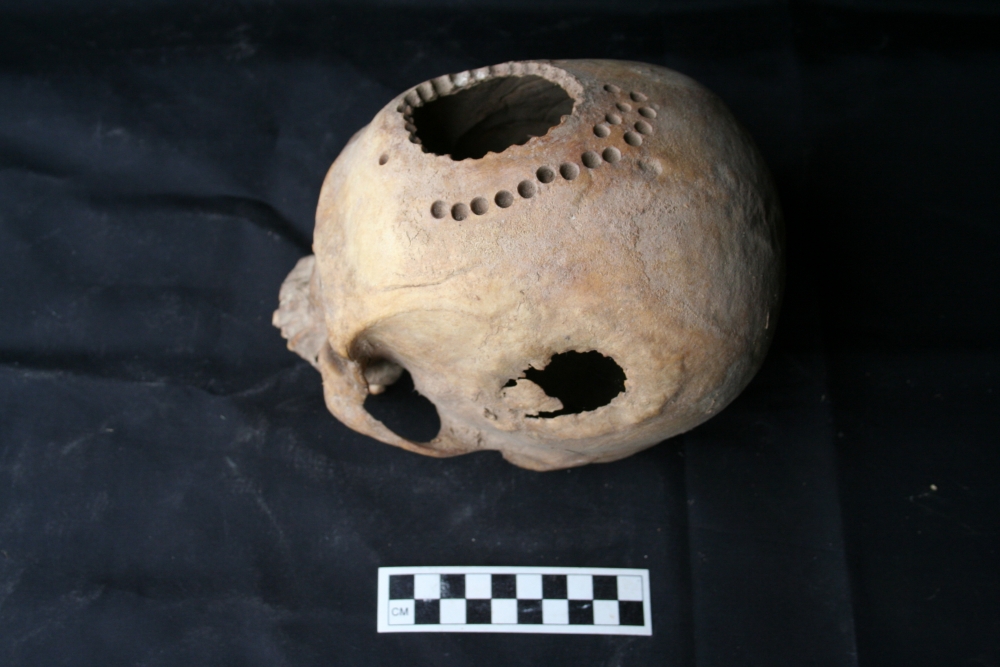The image depicts a mysterious, fossilized artifact that resembles a non-human skull. Positioned on a slightly wrinkled, black cloth of some sort, the fossil is a neutral-toned brown, beige, or tan in color. It features a prominent, scalloped-edged hole at the top and an unusual arrangement of circular indentations, with two lines of smaller circles that seem too precise to be naturally occurring, suggesting they may have been made with machinery. Additionally, there are more jagged and irregular holes at the bottom, giving the appearance of breakage or erosion. For scale, a black and white checkerboard measuring tape marked in centimeters is positioned in the foreground. This specimen likely comes from an ancient life form and may have been unearthed by archaeologists.